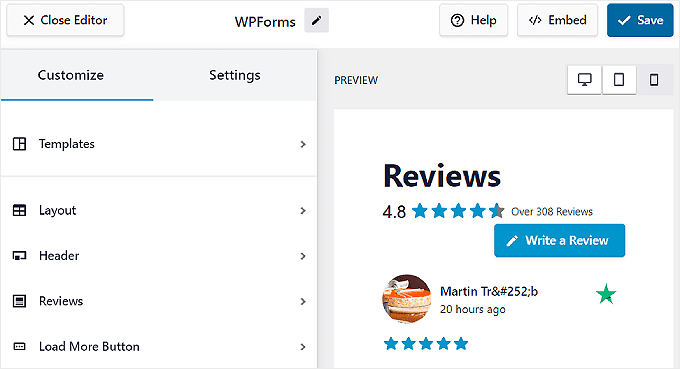In this image, we observe a user interface with multiple layout elements, seemingly part of a design or editing tool for web pages. 

**Upper Left Corner**: There is a "Close Editor" button.

**Top Center**: A header labeled "WPForms" accompanied by a small icon possibly meant for drawing or editing. Next to this header are a "Help" button, an "Embed" button, and a highlighted "Save" button in blue.

**Main Content Area**: The main focus is a preview of a Reviews page. This page features the following:
- **Title**: "Reviews"
- **Rating Information**: Displays "4.8 stars" based on "over 308 reviews."
- **Call to Action**: A button labeled "Write a Review."
- **Review Example**: A detailed review from "Martin, TR," with the identifier "#252B" posted "20 hours ago," rated "5 stars."

**Left Sidebar**: There are sections labeled "Customize," "Settings," "Templates," "Layout," "Header," "Reviews," and a "Load More" button. 

**Styling**: The design has a clean and minimalistic look with a primary color scheme of white and gray, and black text.

Overall, this interface seems to be a page builder or form editor that allows users to design and manage various elements for web pages, specifically tailored for creating review pages.